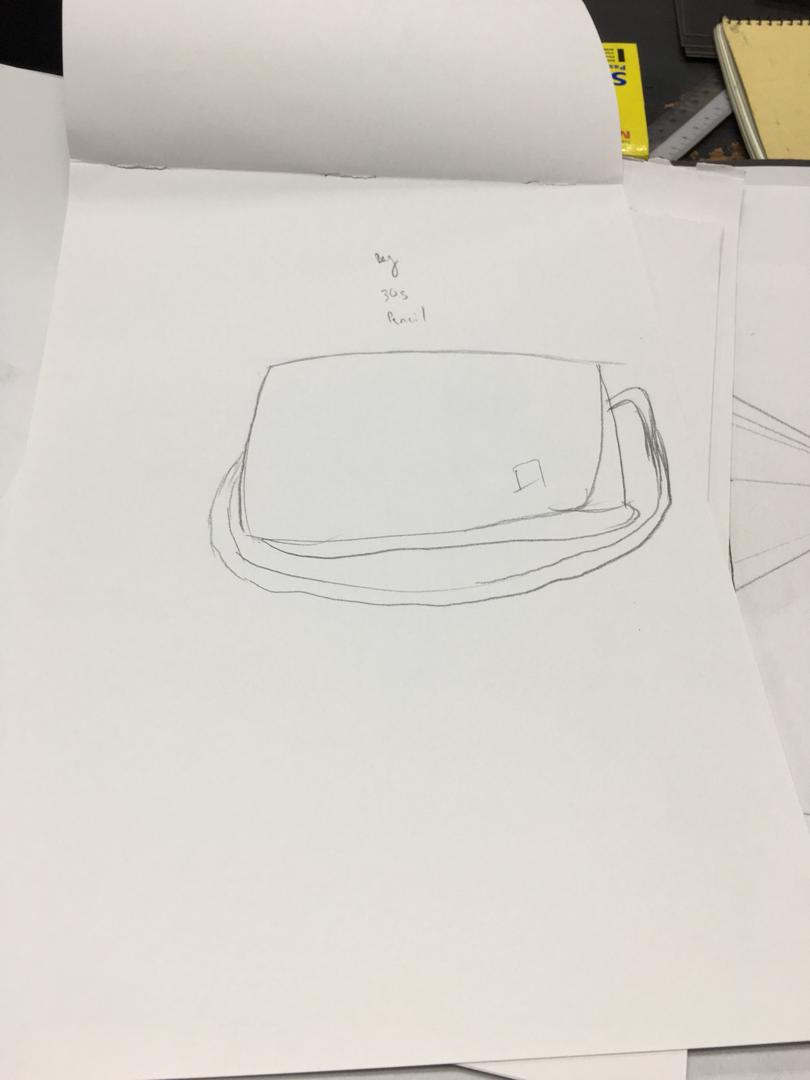The image is a detailed photograph of an open sketch pad displaying a pencil sketch of a handbag. The sketch pad page, which is white and oriented in portrait mode, holds a meticulously drawn handbag with a rectangular shape and a front flap, complemented by a handle or strap that curves underneath the bag's body. Above the bag, the words "bag," "305" or "30S," and "pencil" are inscribed in small text. Beneath the visible page, two other pages of similar size slightly peek out to the top right, and near the bottom right corner is another torn page showcasing an indeterminate pencil sketch of a triangle extending out of the frame. In the top right corner of the photograph, there is a closed, spiral-bound sketchbook with a vibrant yellow cover. Behind the sketchbook, a metal ruler is visible, accompanied by a packet, likely containing pens or pencils, marked by a yellow cover and blue text.